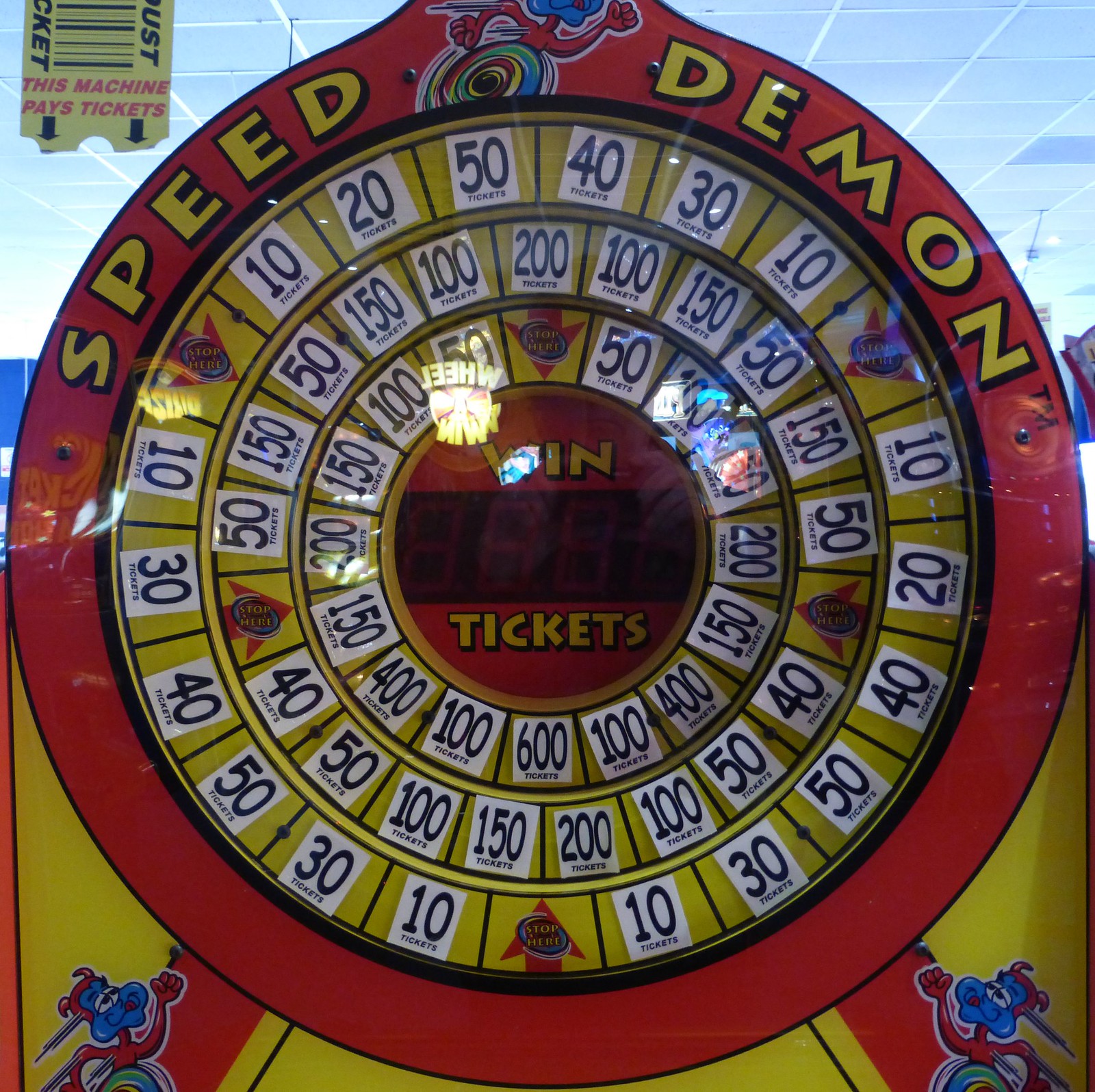The image captures the top section of an arcade game designed to resemble a colorful, interactive gambling machine. Dominating the scene is a large red circular border with the text "Speed Demon" emblazoned in vibrant yellow at the top. Encircling the central point where a digital display screen reads "Win Tickets," are three progressively smaller concentric rings, each filled with various numerical values indicating ticket rewards. 

The outermost ring is decorated with numbers such as 10, 20, 30, 40, and 50, repeated along the circumference. The middle ring showcases higher values like 50, 100, 150, and 200, while the innermost circle boasts even more significant amounts, with numbers reaching up to 600. Scattered around the circles are whimsical cartoon characters resembling small demons or snails with blue heads, adding a playful touch to the game's aesthetic.

A ticket stub positioned nearby states that the machine pays out tickets, emphasizing the game's reward system. This entire setup is set against a white ceiling within an indoor gaming room environment, suggesting a lively, vibrant atmosphere where players can try their luck to win tickets.